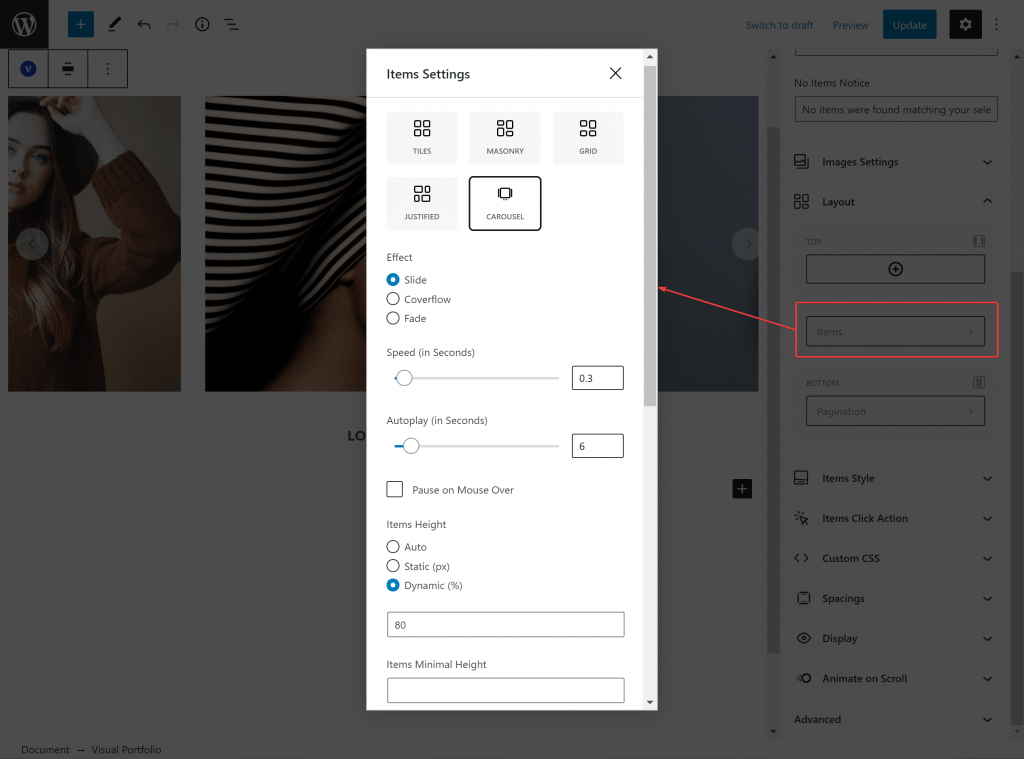The screen displays what appears to be a shopping website, though much of the page is obscured by a white menu overlay. This menu offers various settings for customizing item presentation. Options available include adjusting effects such as "Soft Slide," "Color Flow," and "Fade," as well as setting the speed and auto-play duration in seconds. Additionally, you can specify the item height by entering a numeric value, and set a minimum item height. Upon closer inspection, it becomes evident that this is a web page creation tool designed for configuring the layout and format of an online shopping site.